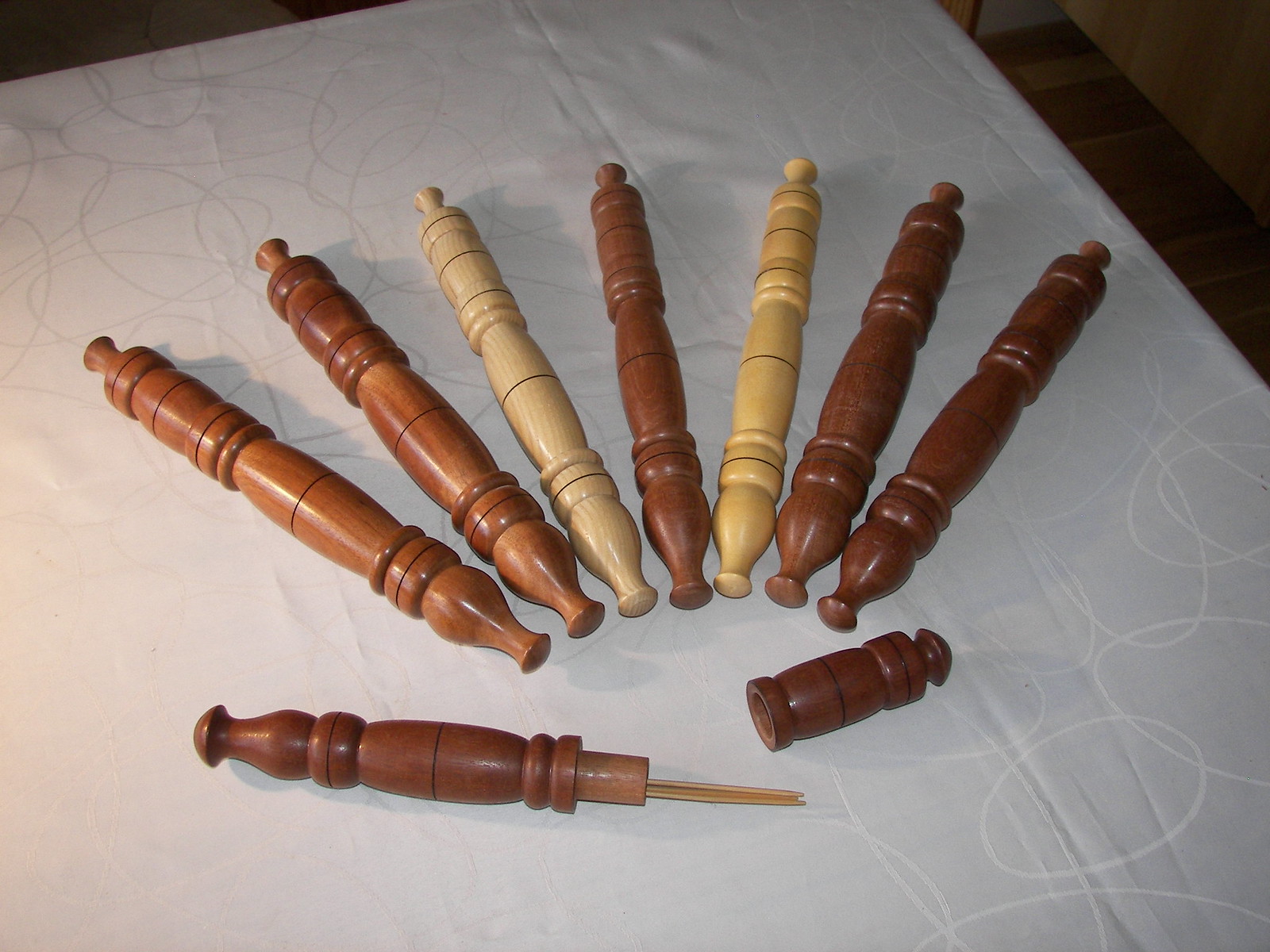This color photograph, taken indoors, showcases eight intricately carved wooden objects, arranged in a visually striking fan-like shape on a white sheet adorned with intersecting ovals. Seven of these spindle-shaped objects, which resemble scroll handles or ornate bed posts, are positioned in parallel, emphasizing their smooth craftsmanship and varying wood stains—from rich dark browns to lighter brown hues. The eighth object, which lies in front of the others, is disassembled into two pieces, revealing a thin stick protruding from one part and a shorter piece lying beside it, reminiscent of incense sticks emerging from their holders. Detailed notches and grooves along the objects add texture and highlight their polished finish, creating an elegant display of traditional woodworking.